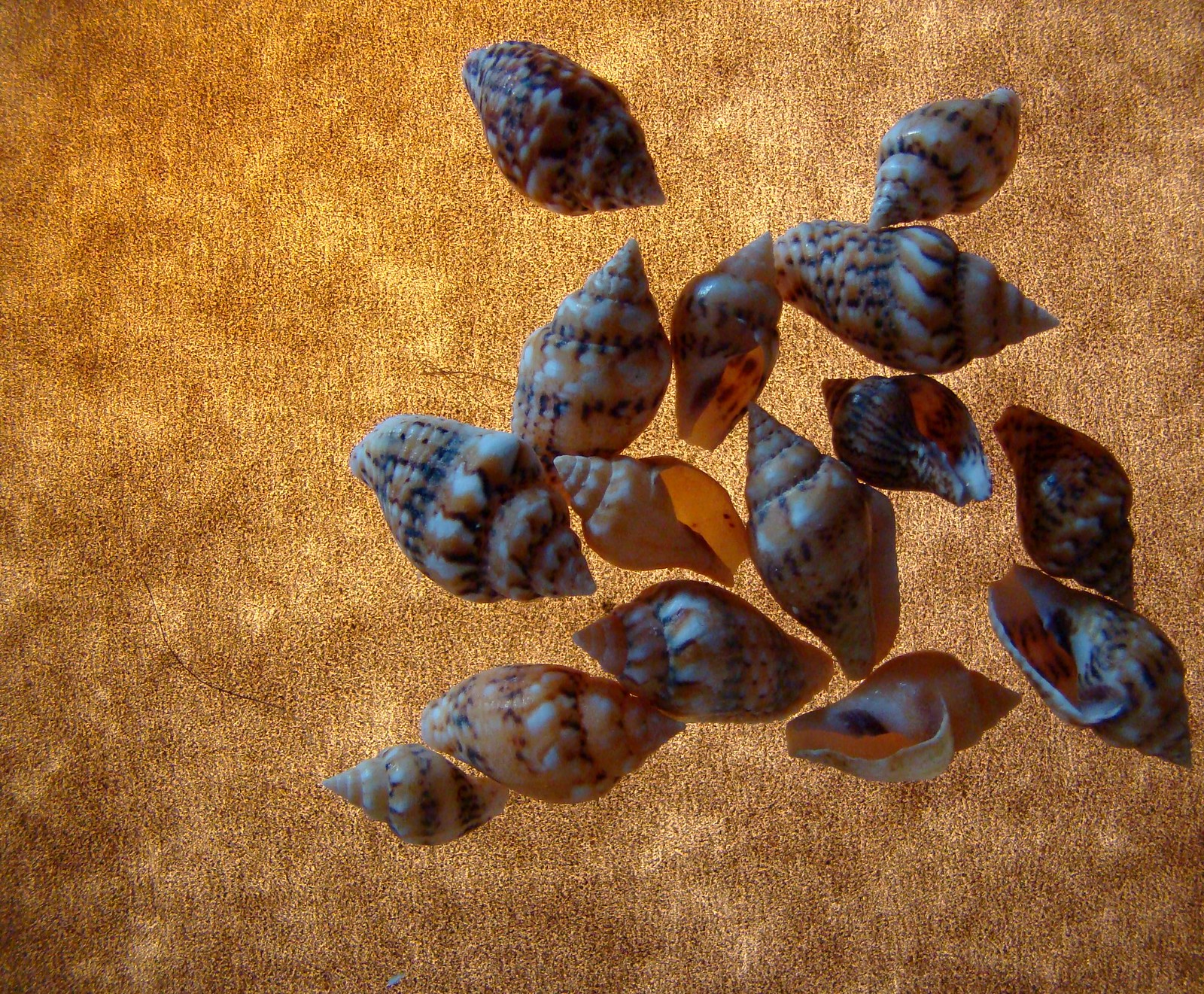The image features around 15 periwinkle shells arranged in a seemingly haphazard pile. The shells, ranging in color from light brown, black, yellow, white, to peach, create a visual contrast against a textured brown background that resembles leather, parchment paper, or possibly carpet. The background exhibits a gradient with a lighter tone in the top left corner, transitioning to a darker hue towards the bottom right. The shells, reminiscent of those that one might hold up to hear the ocean, are smaller and could fit in the palm of your hand. Some shells have their openings visible, offering a glimpse inside, while others display their smooth exteriors. The shells appear to dominate the composition, with a peculiar lighting effect that makes them seem as if they are floating above the background, contributing to a 3D appearance. The arrangement starts with a couple of shells at the top, followed by clusters of three, five, and another five, showcasing both the front and back sides of the shells.